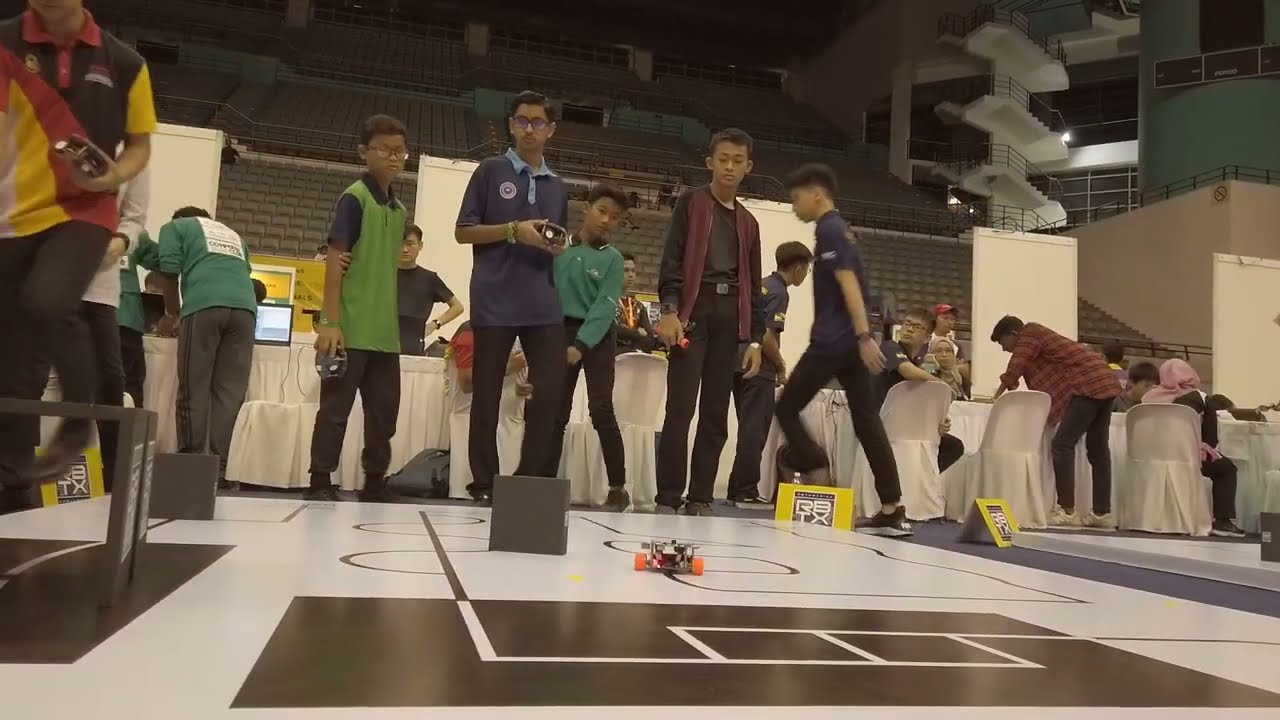This detailed image depicts a lively scene at a robotics competition held in an auditorium or gymnasium. The expansive room features at least three levels of stadium seating stretching up toward the back and to the right, where a set of spiral stairs is visible. Across the back of the photo, a lengthy banquet table spans from left to right, draped in a white tablecloth and lined with matching white-covered chairs. The table seems to serve as a judging area, equipped with laptops and attended by numerous individuals.

In the foreground, five dark-skinned boys of Indian descent, presumably part of a robotics team, are engaged with an activity on the floor. The floor itself is marked with various lines, designs, and black and yellow obstacles, likely part of the competition setup. One of the boys, wearing a gray shirt, appears to be operating a remote control to maneuver a remote control car they likely built for the event. Other participants and attendees can be seen scattered around, either engrossed in their own tasks or observing the main activity. Signs labeled "RBTX" are positioned on each section of the floor, adding to the official atmosphere of the competition.